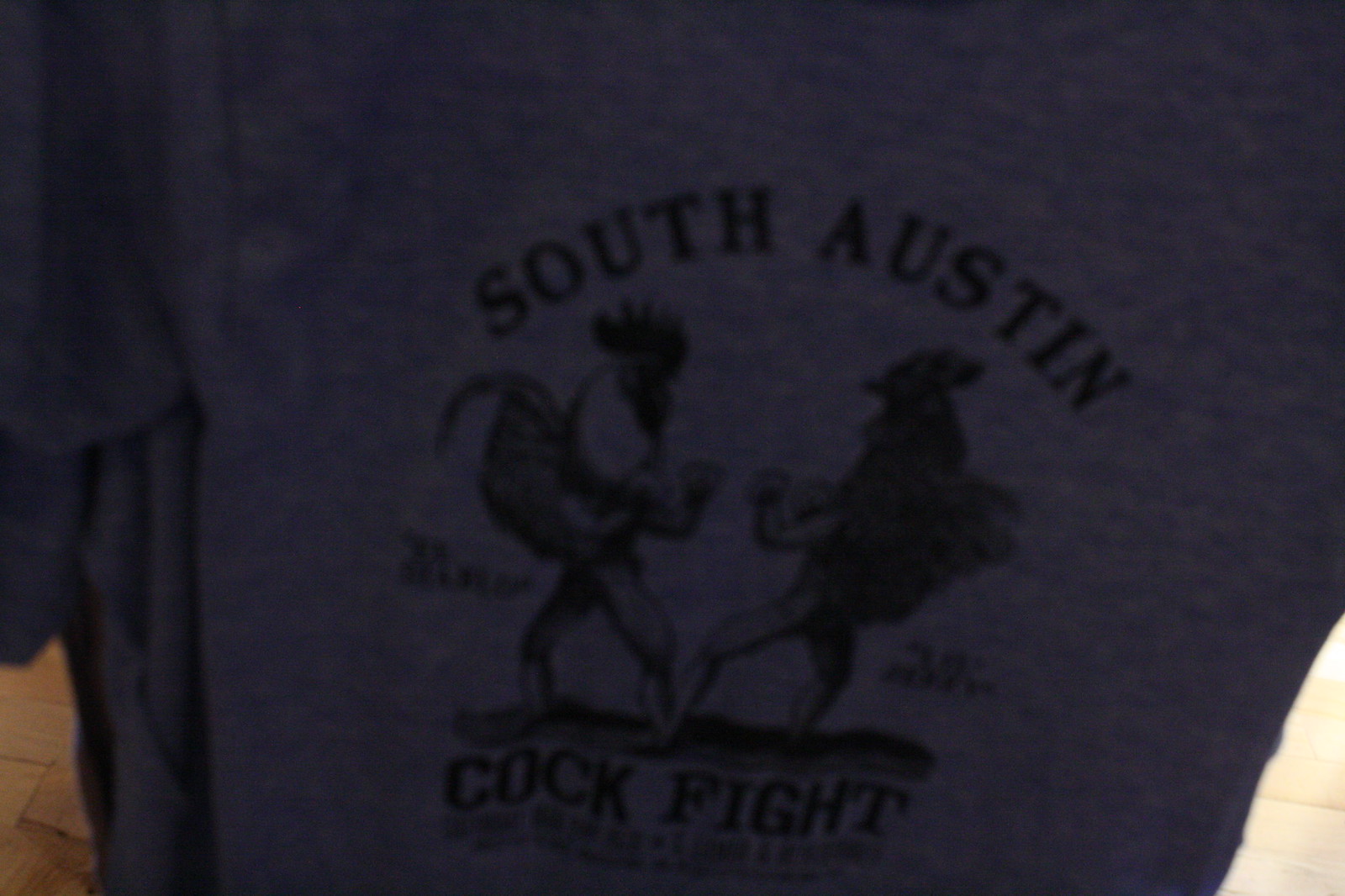This horizontal image captures the front of a t-shirt taken in extremely low light, casting the scene into deep shadows. The hardwood floor background is visible beneath the shirt's arms and around its sides, adding a warm yet subdued texture to the dark setting. The shirt itself features an intense design, almost silhouetted, of two roosters standing on their legs with wings raised as if engaged in battle. These roosters face each other in a combative stance. Above the roosters, arched lettering spells out "South Austin," while the text at the bottom of the shirt reads "Cockfight," framing the fierce imagery between assertive words.